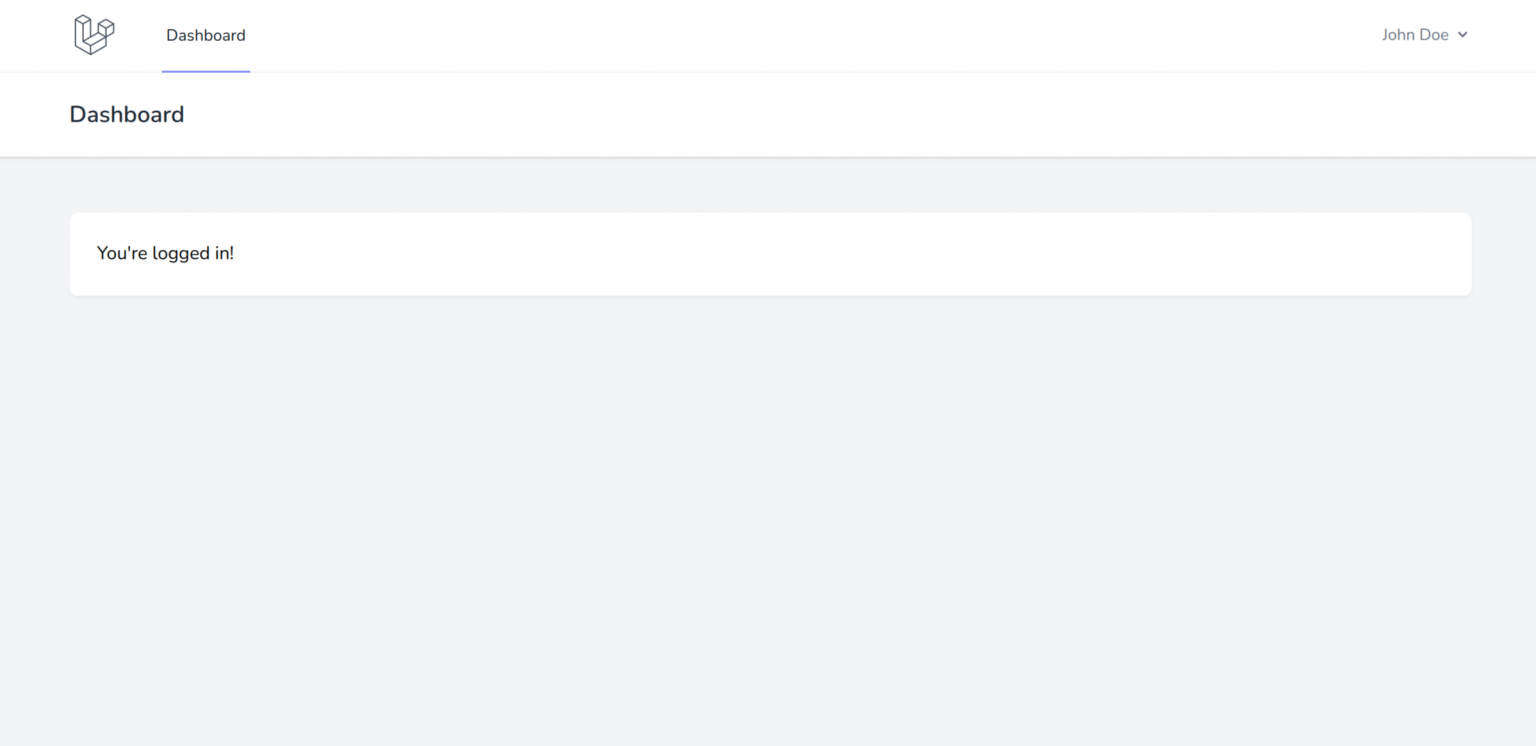The dashboard webpage features a minimalist design with a grey background. At the top, there is a logo consisting of interconnected square shapes, symbolizing the company's visual identity. Next to the logo, the word "Dashboard" is prominently displayed with a distinctive purple underline.

Beneath this header, you find the text "Dashboard" again, followed by the name "John Doe" accompanied by a small grey dropdown arrow, suggesting additional user options.

A white rectangular text box spans across the screen, containing the black text: "You are logged in!" The overall webpage is spacious, dominated by neutral colors and sparse text. One notable visual element is an image resembling a cylindrical structure made up of interconnected blocks, which appears to be the company logo. The design is clean and focused, emphasizing functionality with minimal distractions.